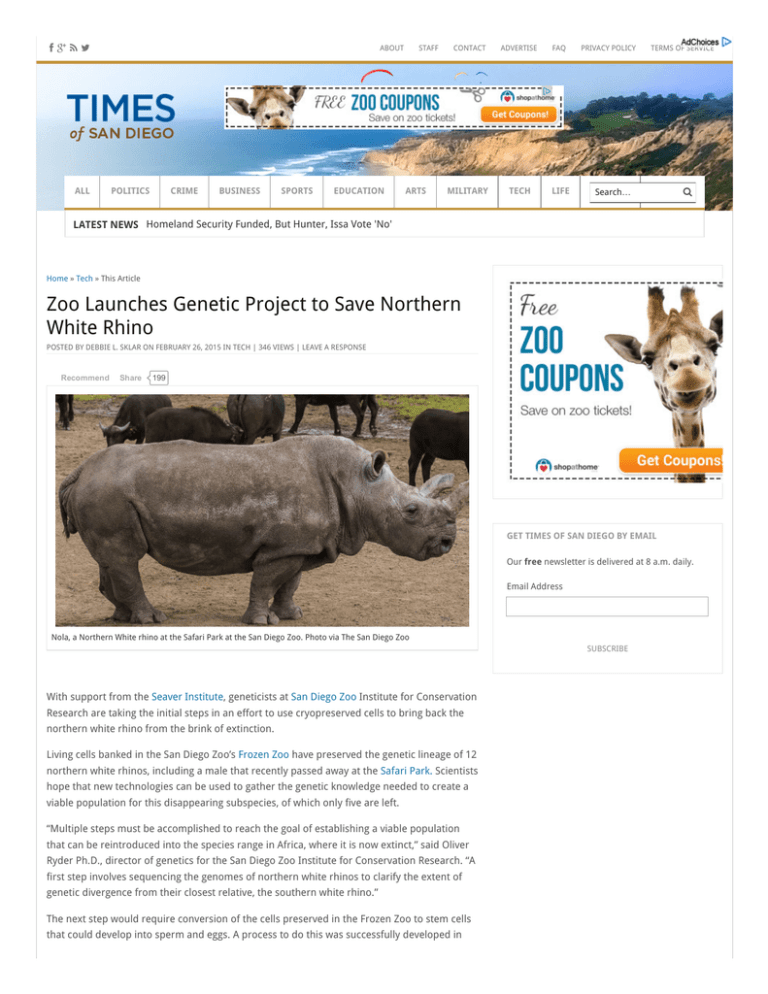The "Times of San Diego" website is neatly organized with numerous navigational features and content areas. At the top, the left-hand corner houses quick access links to social media platforms such as Facebook and Twitter, alongside a Wi-Fi signal icon. On the opposite end, a series of dropdown menus appear, labeled as About, Staff, Contact, Advertise, FAQ, Privacy, Health, and Terms of Use.

Beneath this top navigation bar, a captivating image of a rock cliff overlooking the ocean stretches across the page, enhancing the visual appeal. To the left of this picture, the "Times of San Diego" logo signifies the website's focus on news relevant to the San Diego area.

Below the logo, a second layer of navigation includes selectable tabs for All, Politics, Crime, Business, Sports, Education, Arts, Military, Tech, and Life. Aligned with these tabs is a search bar on the far right for easy information retrieval.

The current screen focuses on the latest news updates, with highlighted stories on Homeland Security funding, a Hunter ISS vote, and more. The user has selected the Home and Tech categories, focusing on an article titled "Zoo Launches Genetic Project to Save Northern White Rhino." Accompanying the article is an image of a Northern White Rhino, followed by several paragraphs of informative text.